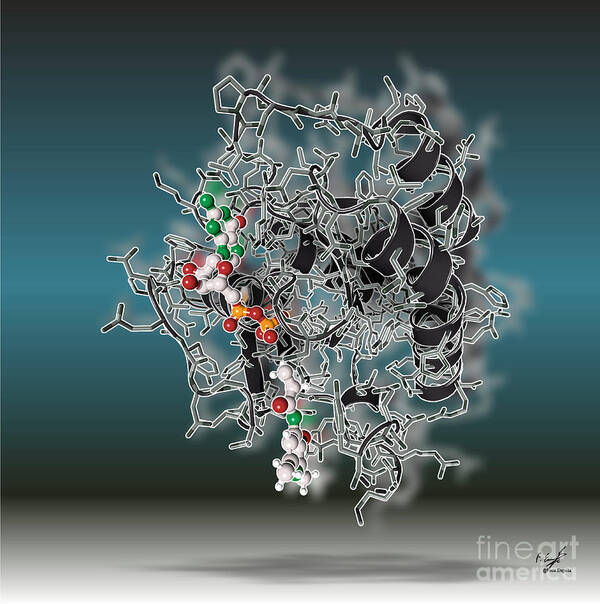The image portrays an abstract art piece with a complex web of interconnected lines and spheres set against a gradient background that transitions from turquoise blue at the top to dark gray at the bottom. The artwork features a tangled network of gray, black, and white lines that are reminiscent of a scientific depiction, such as molecules or chemical structures. These lines, with ribbon-like curls akin to Christmas ribbon or hair curled with a curling iron, intertwine with spherical nodes in various colors—green, white, red, and orange.

On the left-hand side of the composition, a series of nodules is arranged in a squiggly manner. These include configurations like three white spheres connected to a central white sphere, branching out to shapes where red spheres are combined with white, and eventually leading to arrangements with one orange sphere in the center. There are also clusters of colorful dots, predominantly green, white, red, and orange, creating a visually striking pattern against the blurred backdrop. Fine Art America is clearly marked in white in the lower right corner of the image, grounding the ethereal and scientifically inspired abstraction with a touch of reality.